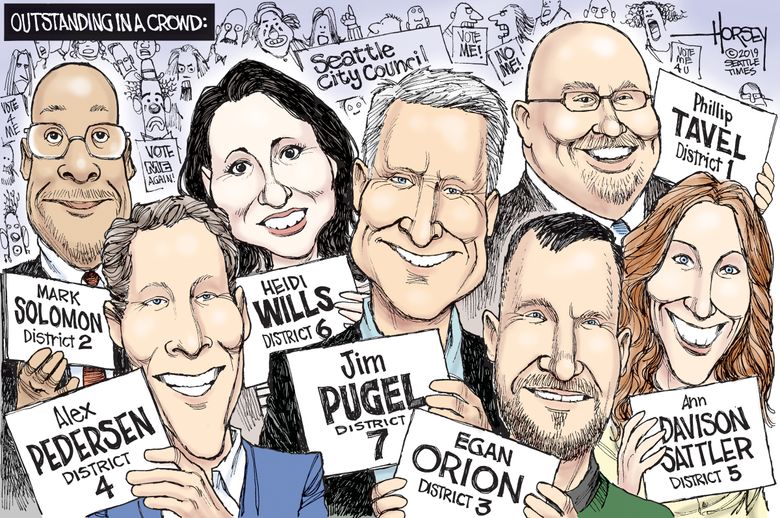The image is a detailed caricature poster titled "Outstanding in a Crowd" in a black rectangle in the top left corner. In the foreground, there are seven caricatured figures, each person holding a white card displaying their name and district number, including Heidi Willis for District 6, Mark Solomon for District 2, Alex Pedersen for District 4, and Jim Poggo for District 7. Each figure has exaggerated, large heads typical of caricatures. In the background, numerous black-and-white caricature figures are holding signs that read phrases like "Seattle City Council," "Vote me again," and "Vote me, no me." The artist's credit, "Horsey Copyright 2019, Seattle Times," is also displayed in the top left corner. The cartoon appears to comment on local Seattle City Council elections, likely requiring familiarity with local politics to fully appreciate the humor.